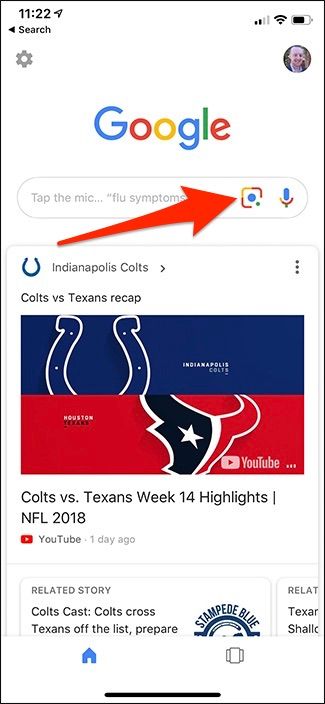The image features a white background with a user interface layout. At the top, there is a search bar displaying the numbers "11:22" with a left-pointing arrow. To the right of the search bar, there is a profile picture of an older man, approximately 60 years old, and next to it is a settings icon.

The central area depicts a Google search interface, highlighted with Google's distinct colored lettering: a blue "G," a red "O," a yellow "O," a blue "G," a green "L," and a red "E." Below this, there is a search bar that includes icons for Google Camera and Google Microphone; a red arrow is specifically pointing at the Google Camera icon.

The main content area features a search result for "Indianapolis Colts vs Texans recap." To the right of the text "Indianapolis Colts," there is an underline symbol ("U") followed by a right arrow and three vertical dots.

Below this, there is a blue rectangle with a white horseshoe, representing the Indianapolis Colts, and a red rectangle depicting a bull's face, half black and half red, symbolizing the Houston Texans. The text "Colt vs Texans Week 14 Highlights NFL 2018" and "YouTube 1 day ago" is prominently displayed.

The image mentions a related story titled "Colts Cast," about crossing the Texans off the list in preparation, though part of the text is cut off. At the bottom of the image, there is a blue house icon within a rectangle.